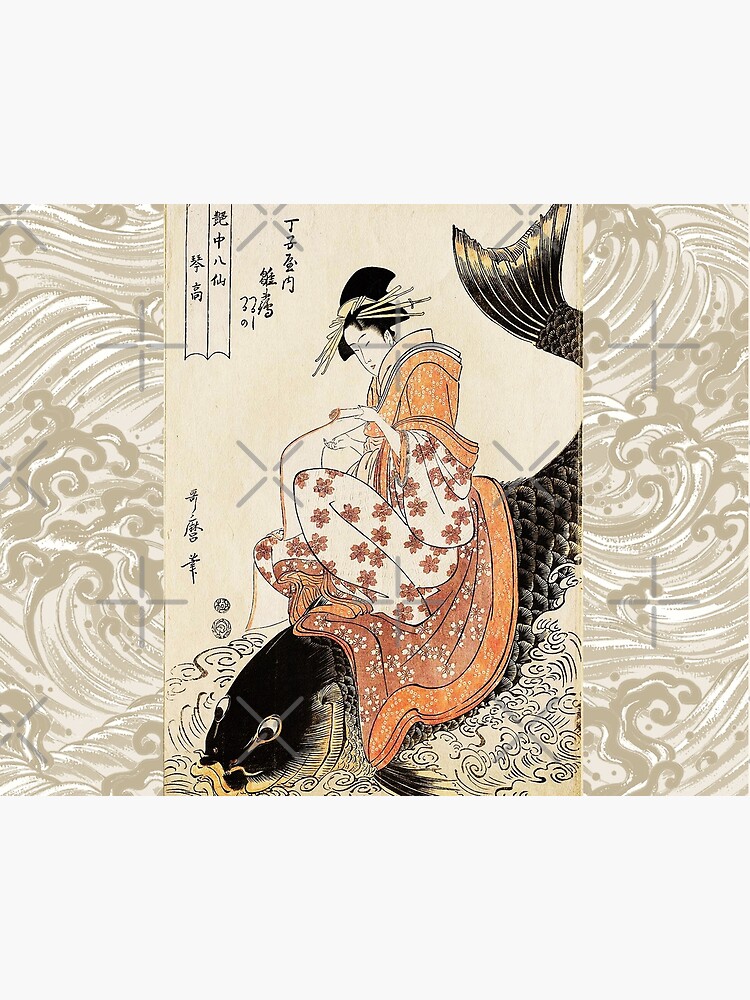This detailed illustration depicts an Asian woman centered against a backdrop of beige light paper adorned with floral and curvy line designs along the edges. The woman, possibly a geisha, has black hair styled in a bun intertwined with straw-like twigs. She wears a traditional orange robe embellished with white and orange flowers and white sleeves. Completing her attire is an ornate mask concealing her face. The woman is seated atop a colossal black fish that features yellow-gold stripes along its back tail, yellow markings near its mouth, prominently scaled body, and large forward-looking black eyes. Surrounding the fish, gray and white wind curls animate the scene, contributing to the dynamic atmosphere. Asian script is present in the upper left-hand corner, adding a cultural and contextual layer to the artwork.